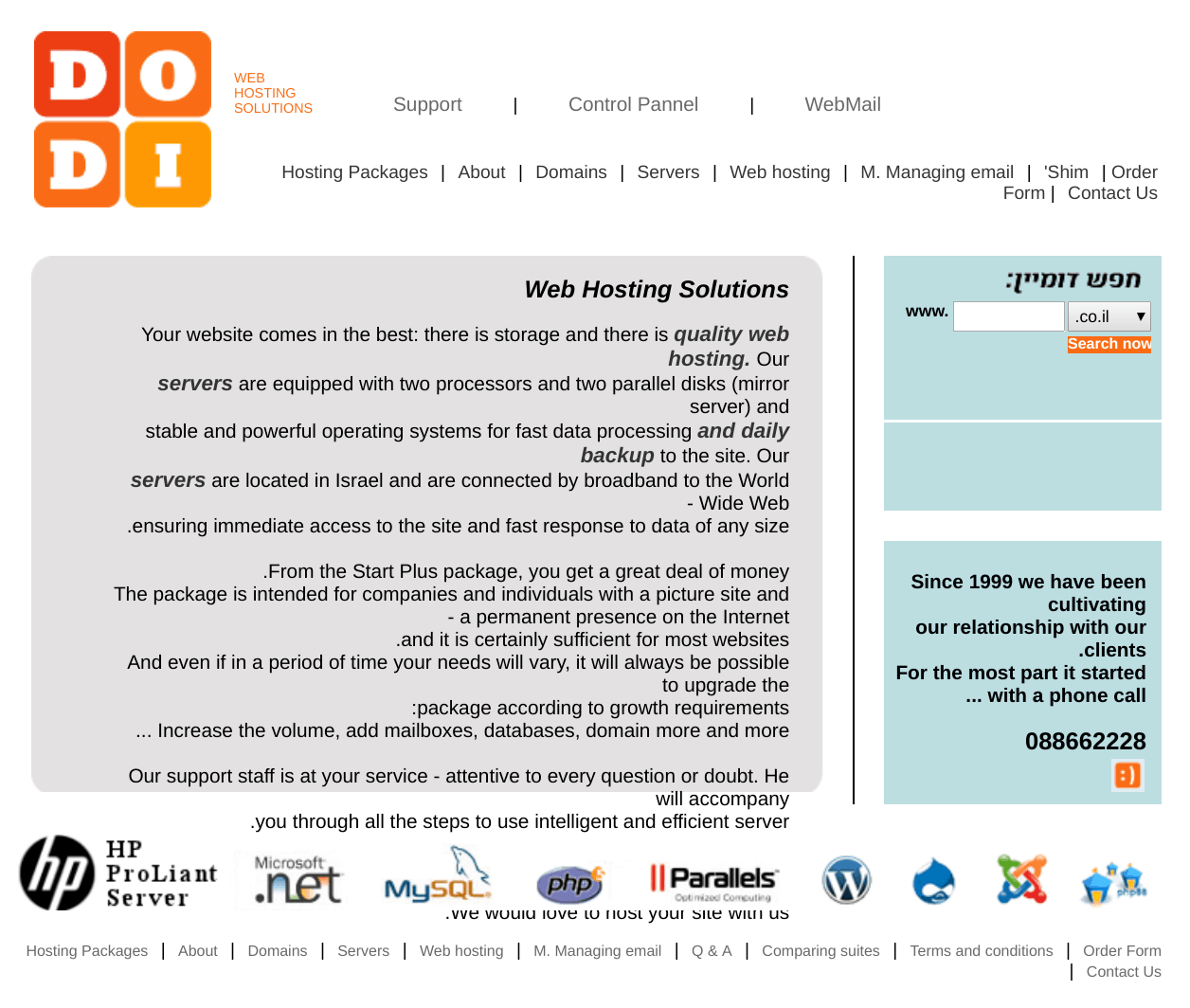This is a screenshot of a website. In the top left corner, there is a logo consisting of four boxes arranged in a cube formation, each containing a single letter. Starting from the top left and moving clockwise, the letters are 'D', 'O', 'I', and 'D'. Next to the logo, there's text in red font that reads "Web Hosting Solutions," followed by text in black font saying "Support - Control Panel," with "Panel" misspelled as "P-A-N-N-E-L," and "/Webmail."

Directly below this header, there is a navigation menu offering several clickable options: "Hosting Packages," "About," "Domains," "Servers," "Web Hosting," "Managing Email," "Order Form," and "Contact Us." 

Beneath this menu, there is a gray square containing text promoting the web hosting services. It reads: "Web Hosting Solutions: Your website deserves the best. We offer storage and quality web hosting. Our servers are equipped with dual processors and two parallel mirror disks, operating on stable and powerful systems designed for fast data processing."